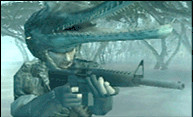The image depicts a small, detailed scene from a fantasy shooting game, showcasing a soldier dressed in a camouflage outfit and khaki, standing more to the left side of the image and facing right. He is holding an assault rifle with a cooling shield, appearing to aim it through the eyepiece with a focused look on his exposed face. Notably, he is wearing fingerless gloves, with the index and middle fingers removed. His headgear resembles an elongated crocodile or alligator head, with its jaws protruding from his forehead. The background has a swamp-like setting, featuring trees typical of such an environment, all tinged in a greenish hue.